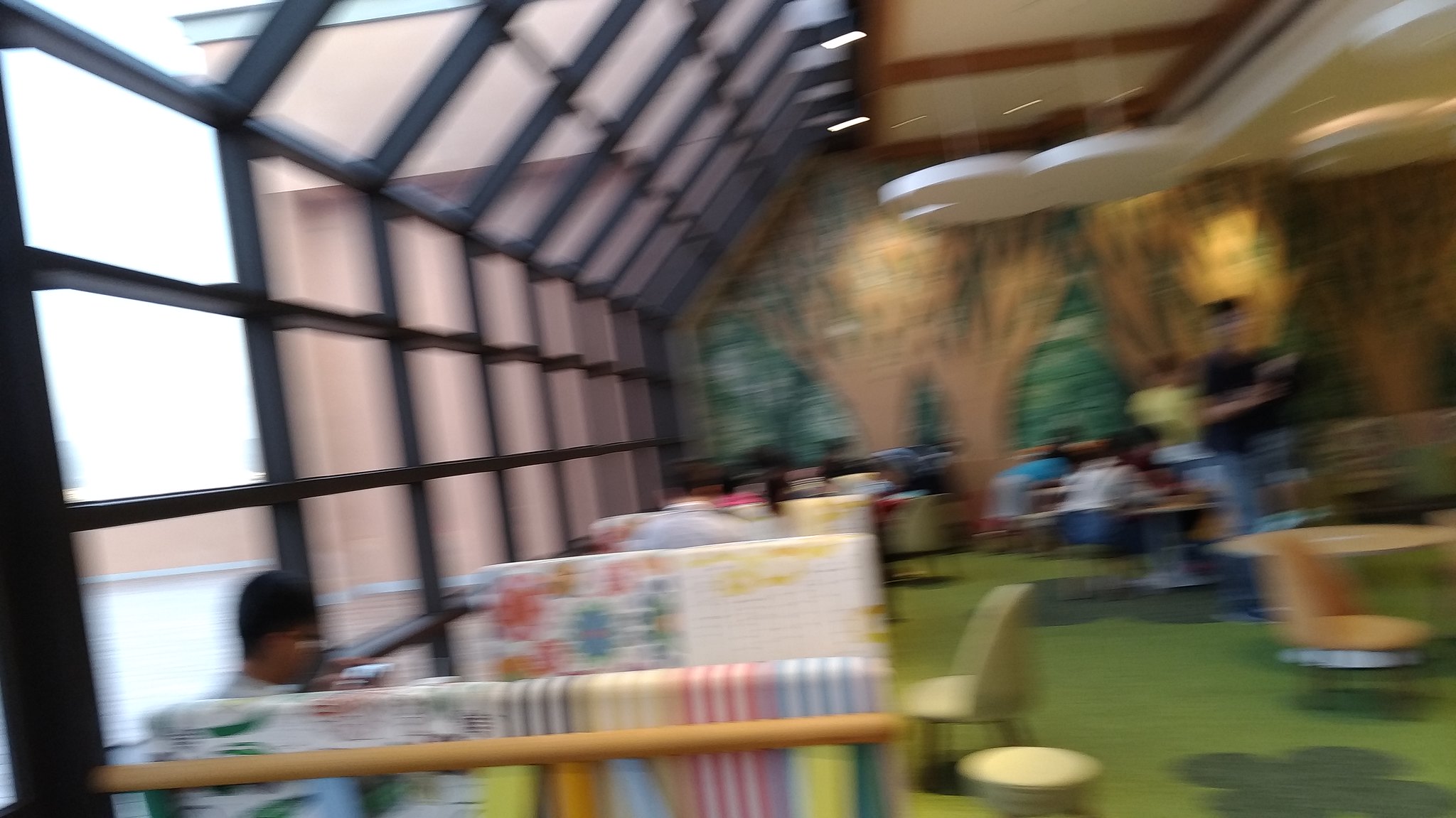A vibrant yet blurry photograph captures the interior of an atrium or sunroom in vivid color. The image is out of focus, suggesting the camera was in motion when the picture was taken. On the left side, a wall of windows allows light to flood the space, perhaps illuminating some seating—likely benches—where a person can be vaguely made out. The back wall is adorned in green, decorated with what appears to be dried grass or painted coral patterns. Dark green carpeting covers the floor, dotted with scattered single chairs. The overall composition is colorful yet indistinct, evoking a sense of movement and a slightly surreal atmosphere.